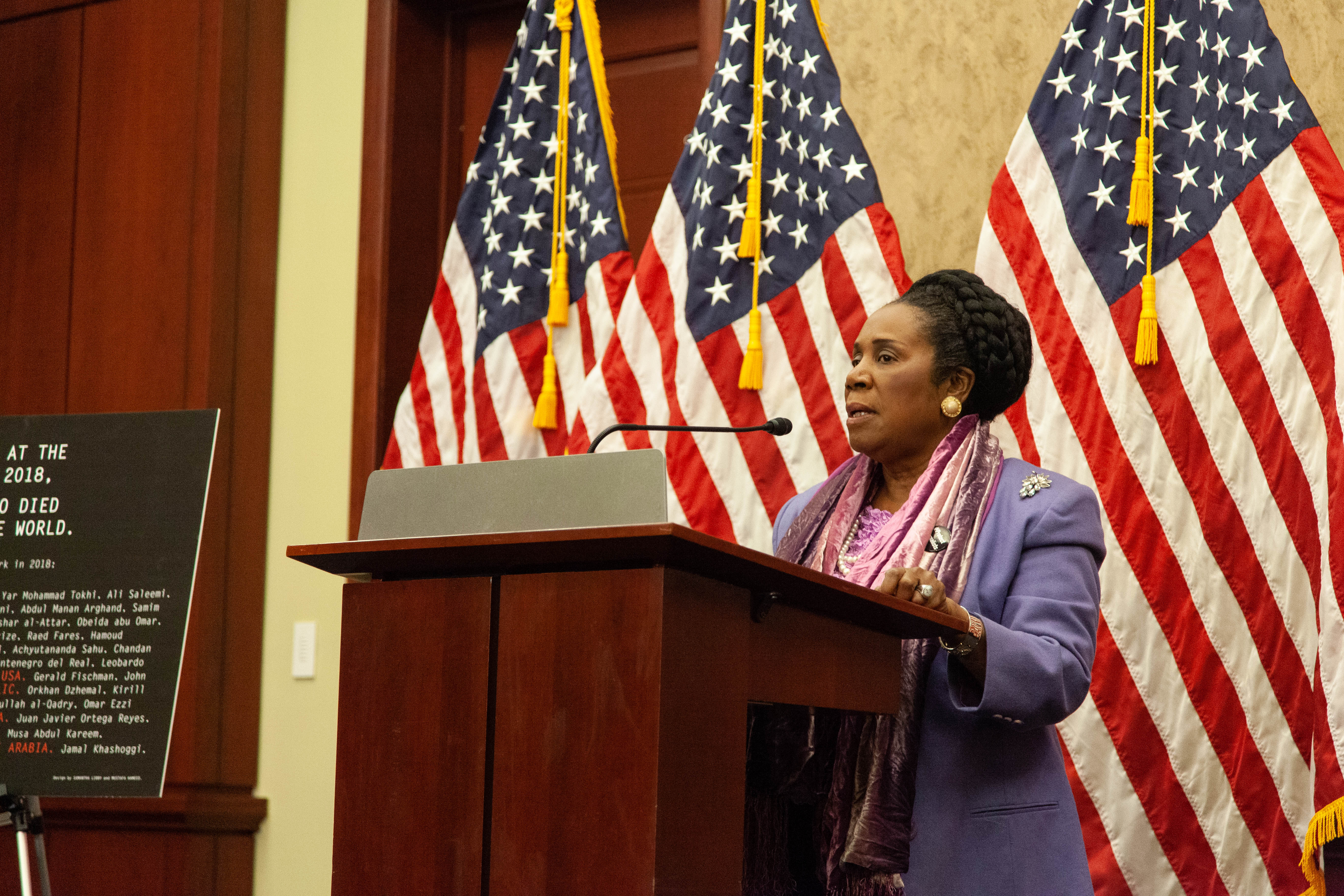The image features a poised black woman, presumably a United States Senator or a member of the House of Representatives, standing at a wooden podium equipped with a microphone. She is dressed in an elegant purple suit jacket adorned with a notable pin and a statement ring. Around her neck, she wears a pink accessory that complements her attire. Her hair is neatly pulled back, highlighting her large earrings. Behind her, three American flags stand prominently against a backdrop of wood paneling. To her left, although partially obscured, there is a sign that remains unreadable. The setting exudes officialdom and a sense of gravitas.